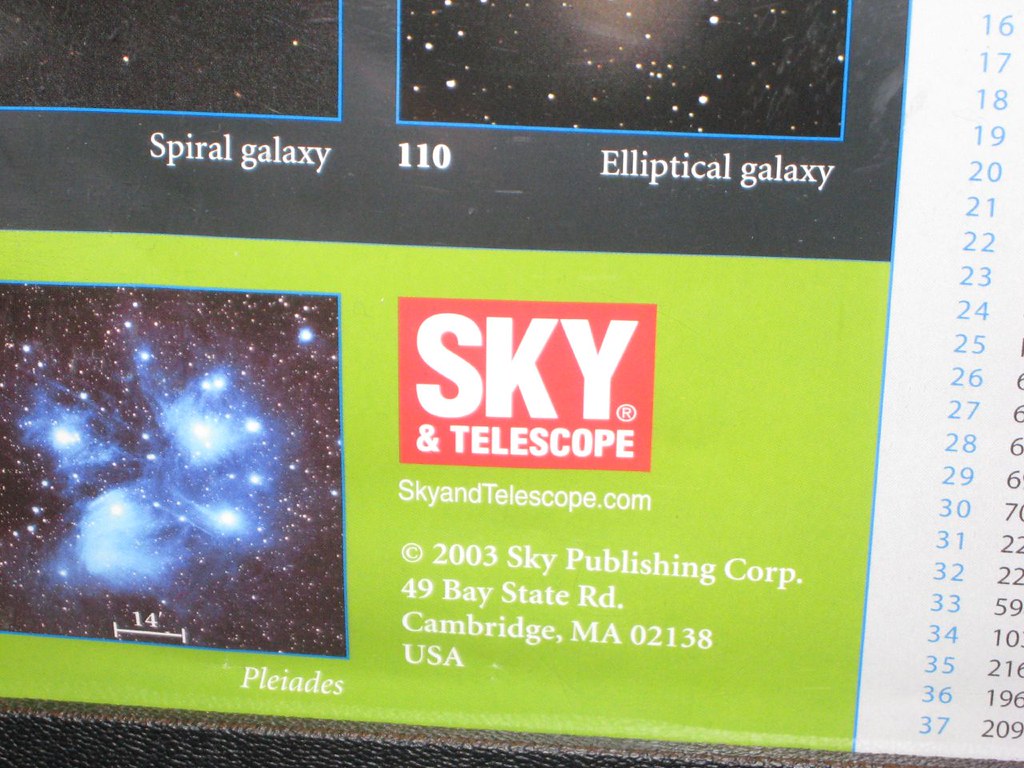The image appears to be a detailed advertisement banner for a telescope company, printed on a board. The top portion features a black background with images framed in blue. To the left is a picture partially visible, depicting stars, labeled "Spiral Galaxy" in white font. Adjacent to it, also framed in blue with visible stars, is labeled "Elliptical Galaxy" in white letters.

Below these, there's a lime green box on the left side, showing a sky scene framed in blue, labeled "Pleiades" in white letters. To the right of this box is a red box with the text "Sky and Telescope" in white, followed by "skyandtelescope.com," and further details including the company's address: "49 Bay State Road, Cambridge, MA 02138, USA." The advertisement mentions "copyright 2003 Sky Publishing Corp." indicating the content and the address information. There are measurements and numbers associated with the images, suggesting the magnification or other relevant details about the telescopes' capabilities.